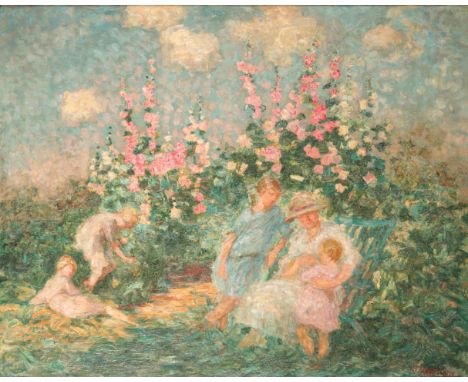This is an early 1900s watercolor painting portraying a serene garden scene. A woman, dressed in a white dress and a tan sun hat, is seated in a chair amidst vivid greenery and colorful flowers. She lovingly holds on to a toddler in a pink dress who leans against her hip. To her right, an older girl in a blue dress stands close, gazing down at the toddler. On the left side, two other young girls, also in pink dresses, are seen picking flowers. The background showcases tall stalks of pink and orangey-pink flowers, set against a backdrop of lush greenery, a blue sky, and fluffy white clouds. There appears to be a small, indistinct signature in the corner of the painting, possibly by a famous artist of that period.